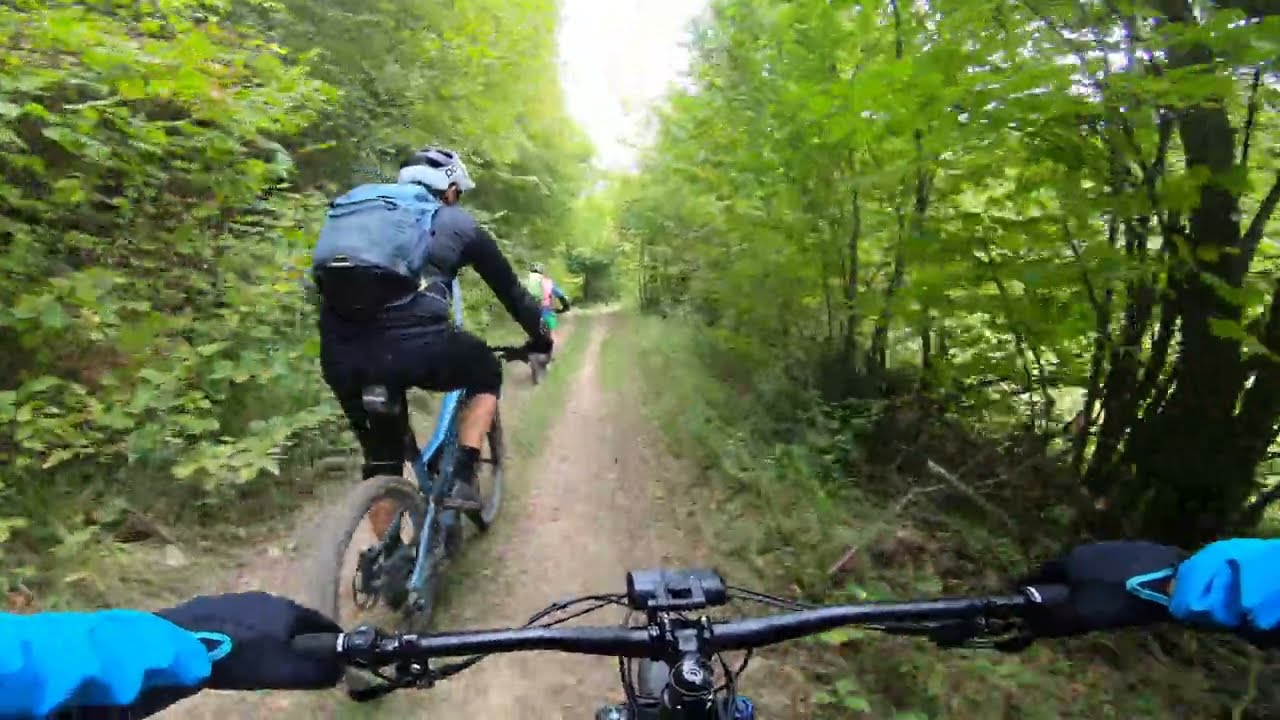This is a horizontally aligned rectangular picture featuring a group of bikers on a narrow dirt trail surrounded by a densely wooded area. At the bottom of the image, in a point-of-view perspective, you see black handlebars with hands gripping them, clad in black gloves and a long-sleeved blue jacket or shirt. The bike's front is partially visible, with the handlebars placed slightly to the right of the trail.

In front of the rider, slightly to the left, is another biker. This person is wearing a tight black outfit, including biker shorts and a top, along with a blue and black backpack. They are riding a blue mountain bike and don a white and black helmet.

Further up the trail, blurred in the distance, is a third rider. This person is dressed in brighter colors, possibly a pinkish shirt and a green backpack, topped with a helmet. The exact color of their bike is indiscernible.

The trail itself is a mix of brown dirt and small patches of grass, with a bit of gravel. The sides of the trail are lined with dense green trees and bright green leaves. The middle to upper part of the image shows a glimpse of bright white sky, suggesting a clear day. The combination of the dirt path, green foliage, and riders create a dynamic and vibrant outdoor scene.